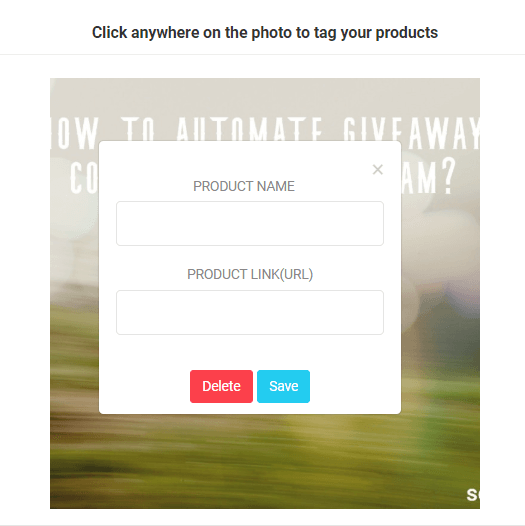In the image, there is a detailed screenshot featuring a predominantly square panel set against a blurred backdrop. The background scene at the bottom showcases vivid green grass transitioning into gray, shadowy bushes or trees. Above, a lighter gray sky with cloud formations is depicted, contributing to the overall hazy appearance, giving an impression of motion from left to right.

The foreground of the screenshot is dominated by large, partially visible white text. Although obscured by a pop-up, the text appears to read, "How to automate giveaway CO... AM?". 

Centrally overlaying the background is a conspicuous white pop-up. The pop-up features fillable fields titled "Product Name" and "Product Link or URL." Both fields are currently empty. In the upper right corner of this pop-up, there is a clickable 'X' symbol to close the window. Below, two buttons stand out: a red "Delete" button and a blue "Save" button. Apart from these elements, there is no additional content visible in the image, emphasizing the function and focus on automating giveaways through inputting product names and URLs.